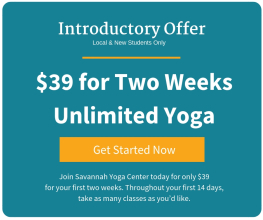Promotional Offer for Savannah Yoga Center

The promotional flyer for Savannah Yoga Center is designed with a teal background and predominantly white text. An introductory offer is highlighted at the top: "Local and new students only: $39 for two weeks, unlimited yoga." Below this offer, an orange "Get Started Now" button stands out, inviting immediate action.

Additional details at the bottom specify, "Join Savannah Yoga Center today. For only $39, enjoy your first two weeks with unlimited access to all yoga classes. Throughout these 14 days, attend as many classes as you'd like." The flyer addresses new students, using the term "students" to refer to its members, reflecting the center's educational approach to yoga. Information on pricing after the initial offer is not provided, leaving potential members to inquire further.